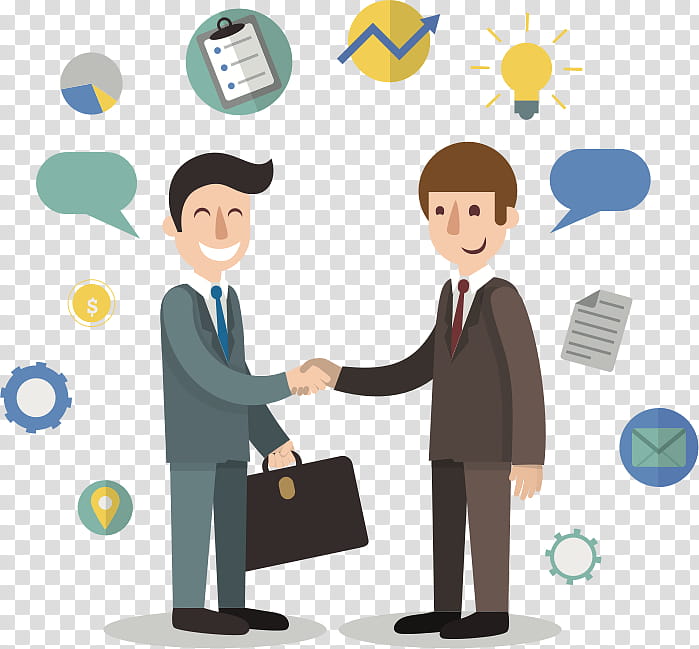In this corporate-themed cartoon image, two men in suits are depicted shaking hands with smiles on their faces, signaling a friendly business interaction. The man on the left, with black pompadour-style hair and dressed in a dark gray suit, white collared shirt, and blue tie, holds a briefcase. The man on the right, characterized by his brown bowl-cut hair and clad in a brown suit, white collared shirt, and red tie, faces his counterpart. Both men are white and their expressions suggest a positive exchange, likely in a business environment. Surrounding them in a circular pattern are various business-related icons, including a light bulb, paper, envelope, map marker, money sign, pie chart, clipboard, stock arrow, and cogwheel, symbolizing ideas, communication, location, finances, analytics, and general business activities. The background is a white and gray checkerboard pattern, emphasizing the clean, professional aesthetic of the artwork. Additionally, speech bubbles are positioned near their heads, indicating a conversation is taking place.